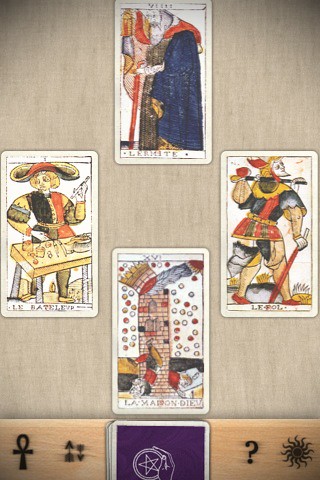The image is a portrait-oriented capture of a digital card game. It is challenging to discern whether it is a screenshot directly from the game or a photograph of a screen. The focal point is a partially visible deck of cards at the bottom, displayed in a traditional portrait orientation but horizontally cut off, only revealing the top halves of the cards. This deck features a purple background and a white border, with the top card slightly misaligned to the right, causing the remaining cards to fan slightly to the left.

The playing area boasts a textured, beige cloth surface with subtle weave patterns and faint darker beige vertical lines that resemble a wood grain. On this surface, four playing cards are arranged in positions reminiscent of the 12, 3, 6, and 9 points on a clock face. These cards are closely packed, overlapping slightly without touching.

Each card is adorned with colorful illustrations depicting characters from a mystical, medieval-like setting. The characters include figures such as wizards, warlords, and jesters, suggesting a departure from traditional playing card suits like hearts or clubs. The artistic detail on the cards highlights the fantasy-themed nature of the game.